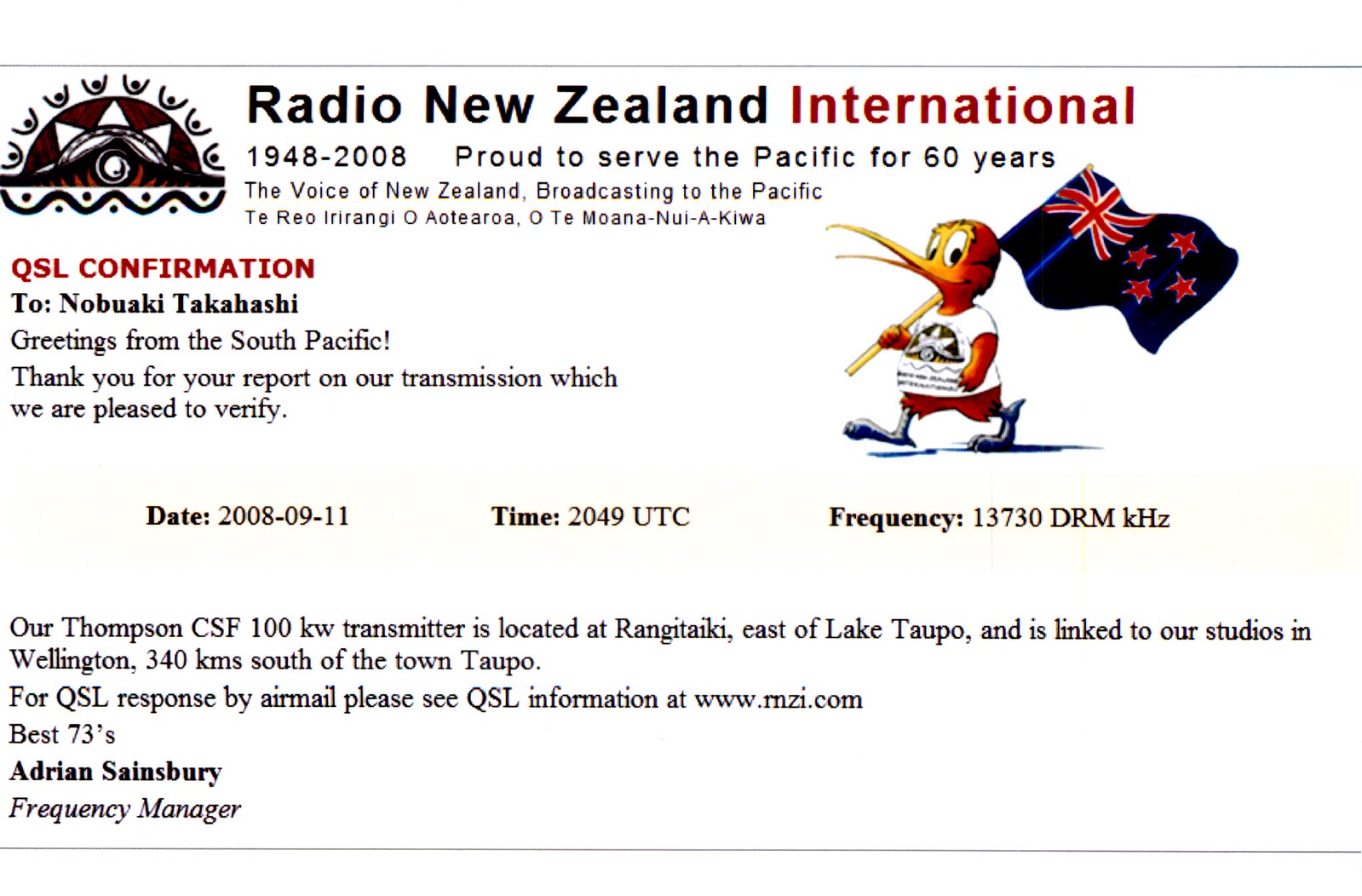The image is an advertisement for Radio New Zealand International, commemorating 60 years of broadcasting from 1948 to 2008. It features a detailed design on a white background with primarily black and red text. The top left corner showcases a logo depicting a sun with an eye, along with waves adorned with dots. Centrally aligned, the text celebrates the anniversary with "Radio New Zealand International, proud to serve the Pacific for 60 years," followed by "The voice of New Zealand, broadcasting to the Pacific" and a line in the Maori language: "Te Reo Irangi Aotearoa o te Moa Nui a Kiwa." 

To the right, there is a cartoon Kiwi bird holding the New Zealand flag, wearing a white shirt with the eye-and-sun logo. Below, there is a QSL confirmation addressed to Nobuaki Takahashi, detailing a transmission verified by Adrian Sainsbury. It records the date as September 11, 2008, the time as 20:49 UTC, and the frequency as 13730 DRM kHz. The message informs that their Thompson CSF 100 kW transmitter is located in Rangitikei, east of Lake Taupo, with its studios in Wellington, 340 km south. For responses via air mail, listeners are directed to visit www.rnzi.com. The advertisement concludes with "Best 73s" and the emphasized name and title of Adrian Sainsbury, Frequency Manager.